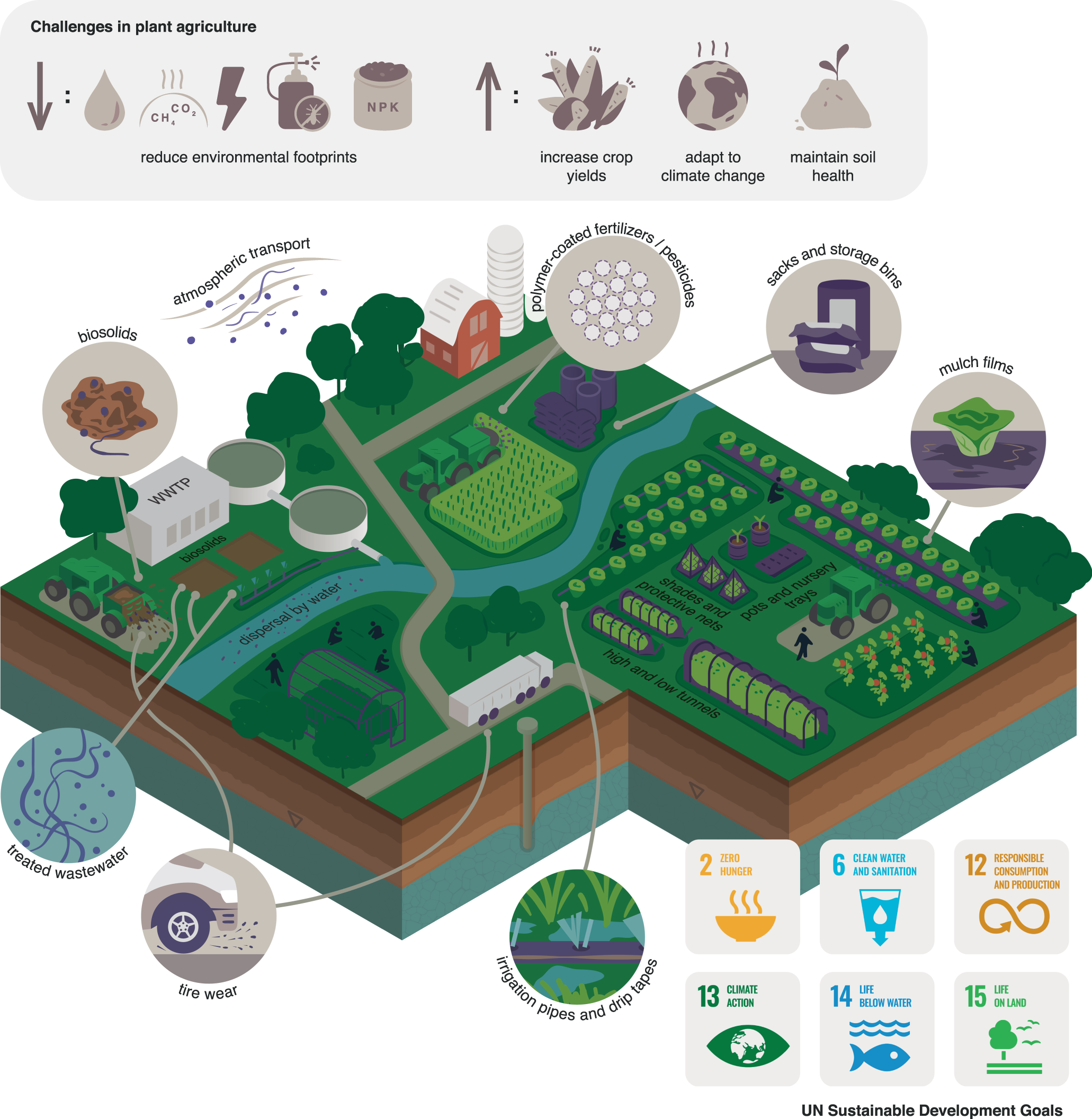The image is a detailed, three-dimensional diagram of a garden complex, illustrating various elements vital for sustainable plant agriculture. The garden plot is fairly large, shown with layers of soil beneath it, and features distinct sections with different plants, including tomatoes and heads of lettuce, as well as a greenhouse. The diagram is busy and rich with information, though most of the text is too small to read clearly. At the top, there is a heading in black that reads "Challenges in Plant Agriculture," accompanied by icons representing increased crop yields, adaptive climate change measures, maintaining soil health, and reducing environmental footprints—depicted with symbols such as water drops and lightning bolts. Additional details include "atmospheric transport" and "polymorph coated fertilizers, pesticides," around the garden area. At the bottom, in very small writing, it mentions the UN Sustainable Development Goals as the source of the diagram. The overall layout resembles a map one might find at an amusement park, guiding through various aspects of agricultural sustainability practices essential for maintaining a healthy, productive garden. Despite the informative nature, the small and illegible text makes it challenging to fully grasp all details at this scale.